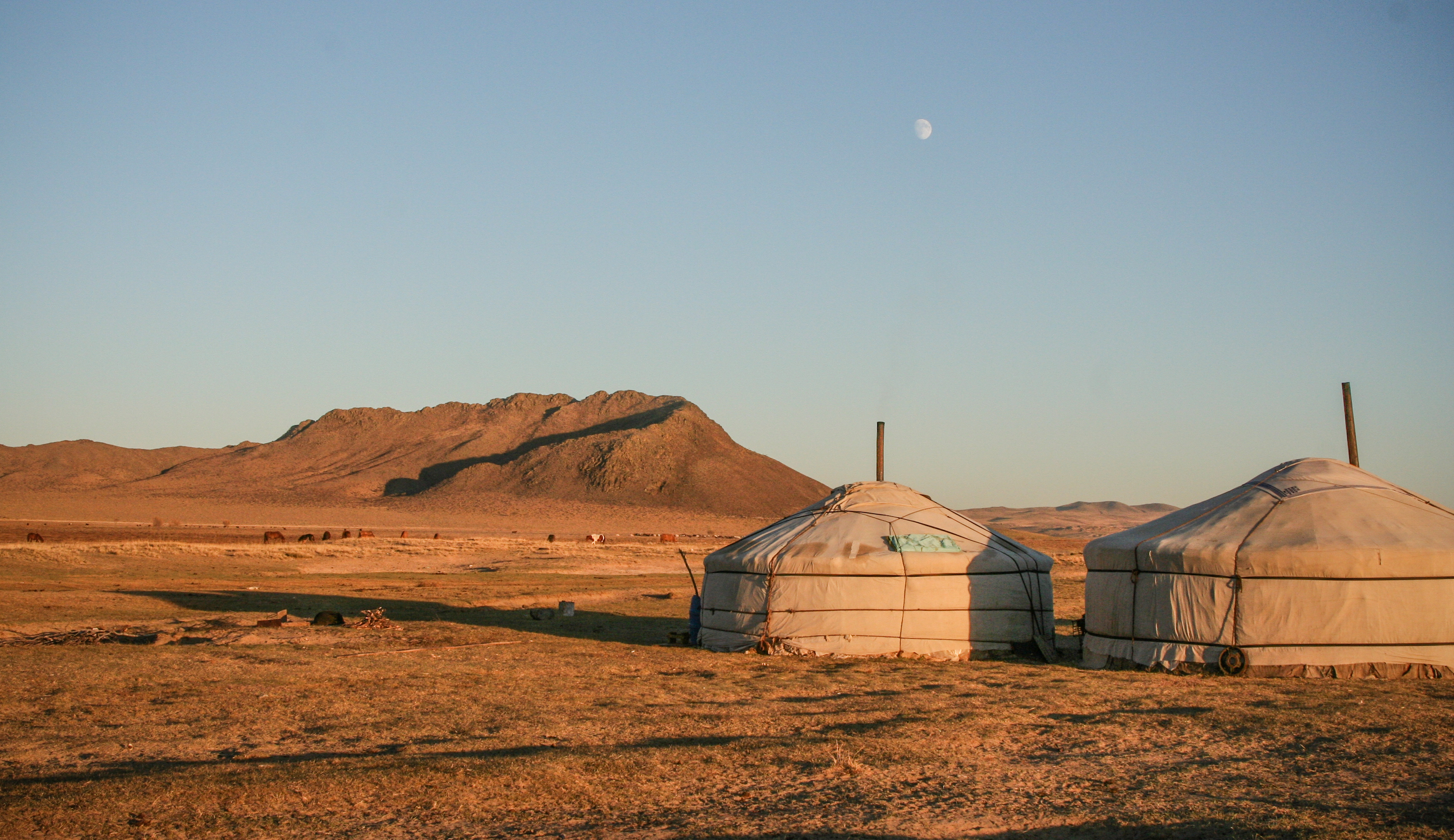The image captures a serene desert or arid grassland landscape under a light blue daytime sky with the moon faintly visible. Dominating the middle ground is a rugged mountain range with brown slopes stretching across the scene. In the foreground, the ground is covered in brown or dead grass, and prominently on the right are two circular tents with a tan hue, resembling traditional Asian or Chinese yurts rather than Native American teepees. These tents are modestly constructed with ropes and central poles. Scattered across the distant background are small figures of livestock, likely cows or perhaps wild horses, grazing peacefully. The vista exudes a sense of dryness and tranquility, devoid of any human presence.